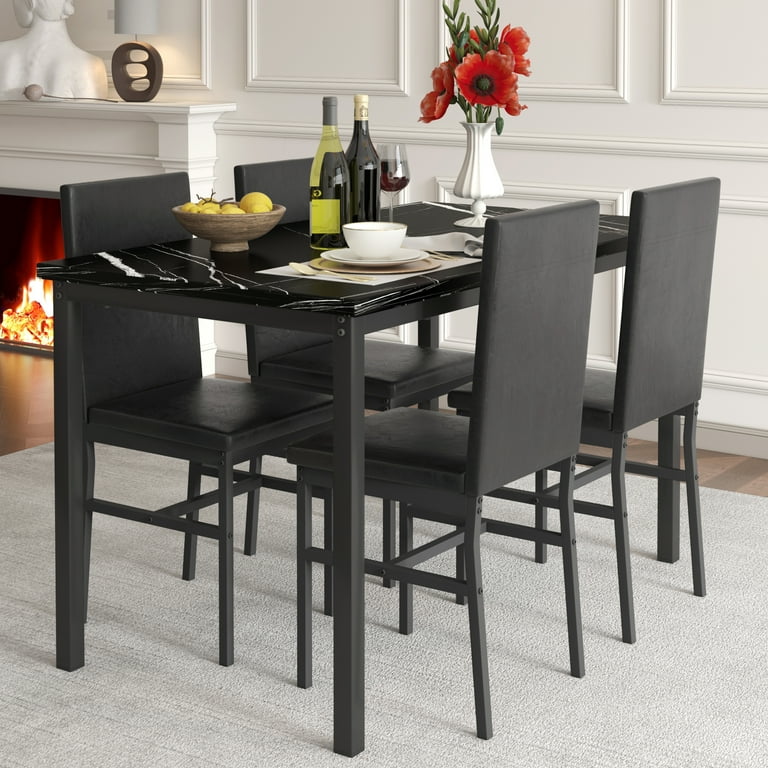In this indoor scene, we have a sophisticated dining room setting featuring a black rectangular table with a black and white marble top, placed on a light-colored rug. The table is paired with four straight, angular black chairs, each with thin, square legs. On the left side of the table, a wooden bowl containing fresh lemons is positioned, while a white vase with vibrant red poppies and green leaves adds a touch of elegance. 

A single place setting includes a light-colored placemat, a brown charger plate, a white ceramic plate, and a white soup bowl. Nearby, there is a partial glass of red wine along with two wine bottles—one likely containing white wine and the other red. The backdrop features a white paneled wall to the right and a cozy, lit fireplace to the left. The fireplace mantle is adorned with a statue and a dark grayish-brown ornament, contributing to the room's modern yet inviting aesthetic. The overall atmosphere of the photograph emanates a clean, luxurious, and curated feel.